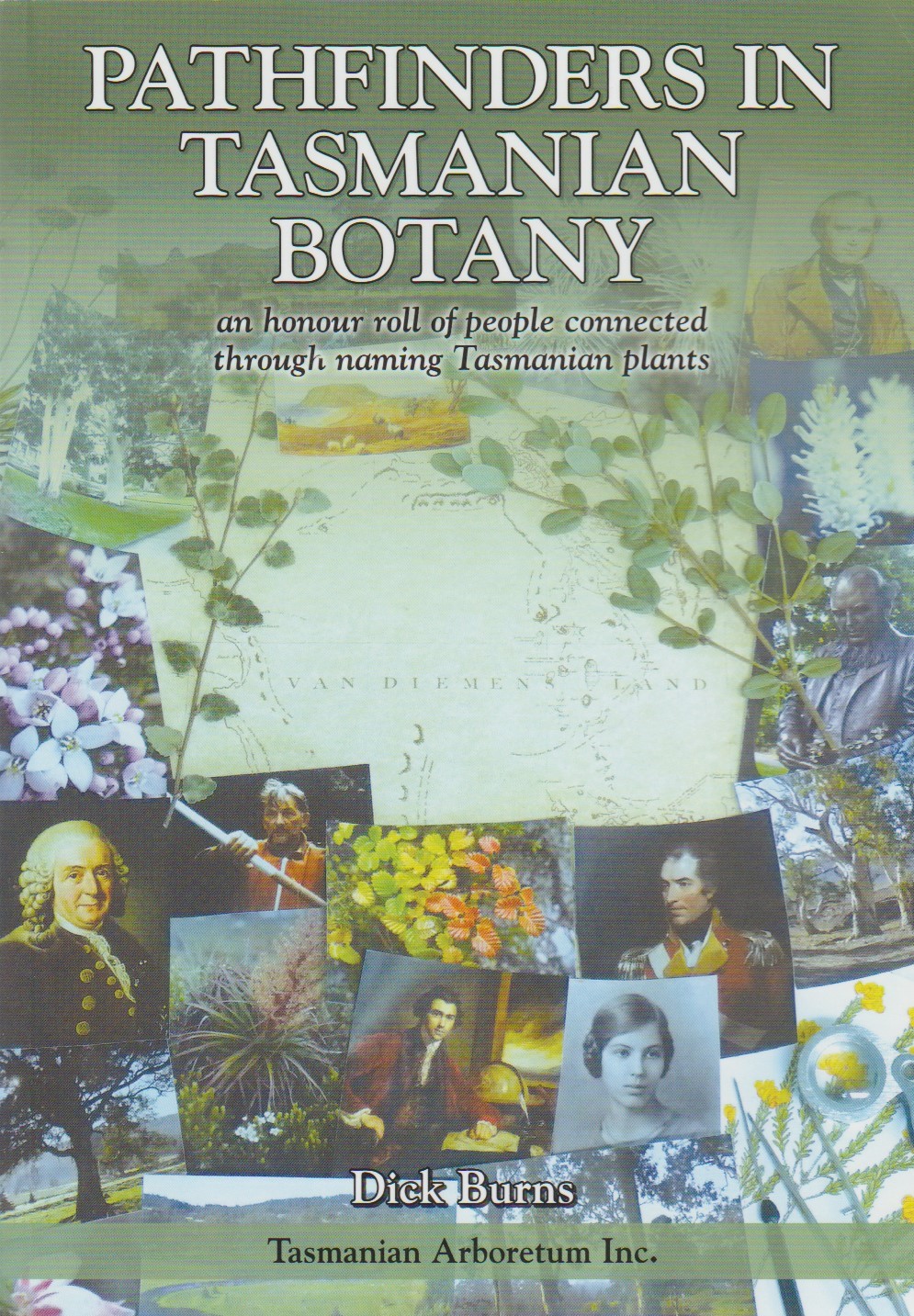The cover image is a collage design for a book titled "Pathfinders in Tasmanian Botany" with a subtitle "An Honor Roll of People Connected Through Naming Tasmanian Plants." The title is prominently displayed at the very top of the cover in white block text, while the subtitle appears below it in smaller black text. The background of the cover gradually transitions from a faded image at the top to more vibrant images towards the bottom, blending a sense of historical depth with modern clarity.

Central to the background is a map, adorned with images of various Tasmanian plants and scattered photographs of people, hinting at their contributions to botany. The people featured include diverse figures such as men and women, captured in both historical black-and-white and contemporary photographs, suggesting a timeline of botanical exploration. Specific images include individuals in military uniforms, a woman with a hair bun, a man at a writing desk, a man potentially in a kayak, and even a statue, creating a rich tapestry of personalities connected to Tasmanian botany.

At the bottom of the cover, the author’s name, Dick Burns, is prominently displayed in white font. Directly underneath, in black text on a green strip, is the mention of "Tasmanian Arboretum Inc.", indicating the likely publisher or associated institution. The overall design, though somewhat busy, effectively conveys the intertwined history of people and plants in Tasmanian botany.